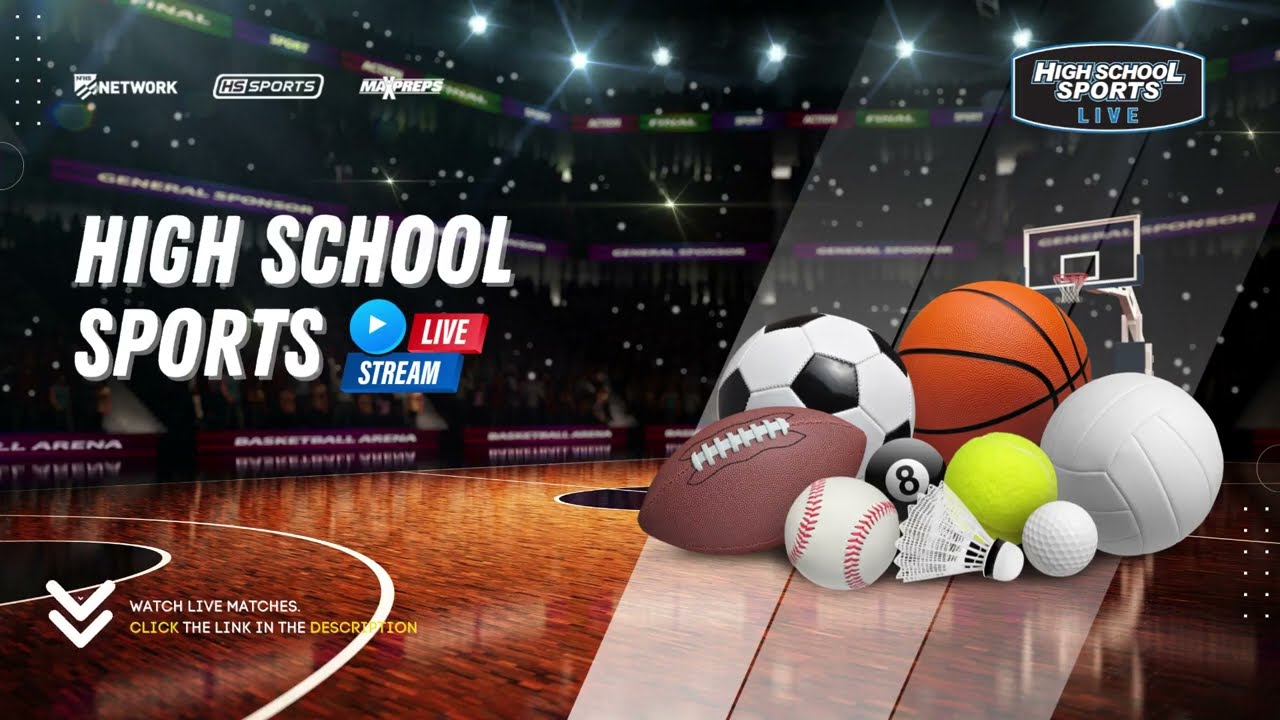The image is a detailed, computer-generated graphical representation of a brightly lit, indoor basketball stadium with multiple audience levels and extended rafters reaching up to the ceiling. On the right side of the court, there is an array of various sports balls including a basketball, soccer ball, tennis ball, baseball, badminton birdie, football, volleyball, an 8-ball, and a golf ball, all illuminated by spotlights from above. White oblique transparent strips run behind the balls, adding a dynamic visual effect. The top right corner of the image features the text "High School Sports Live," while the upper left corner displays "Network HS Sports" and "ML Preps." Beneath this, the text reads "High School Sports Livestream." The bottom of the image has a prompt that says, "Watch live matches, click the link in the description," suggesting it is an advertisement for a live stream service for high school sports events.